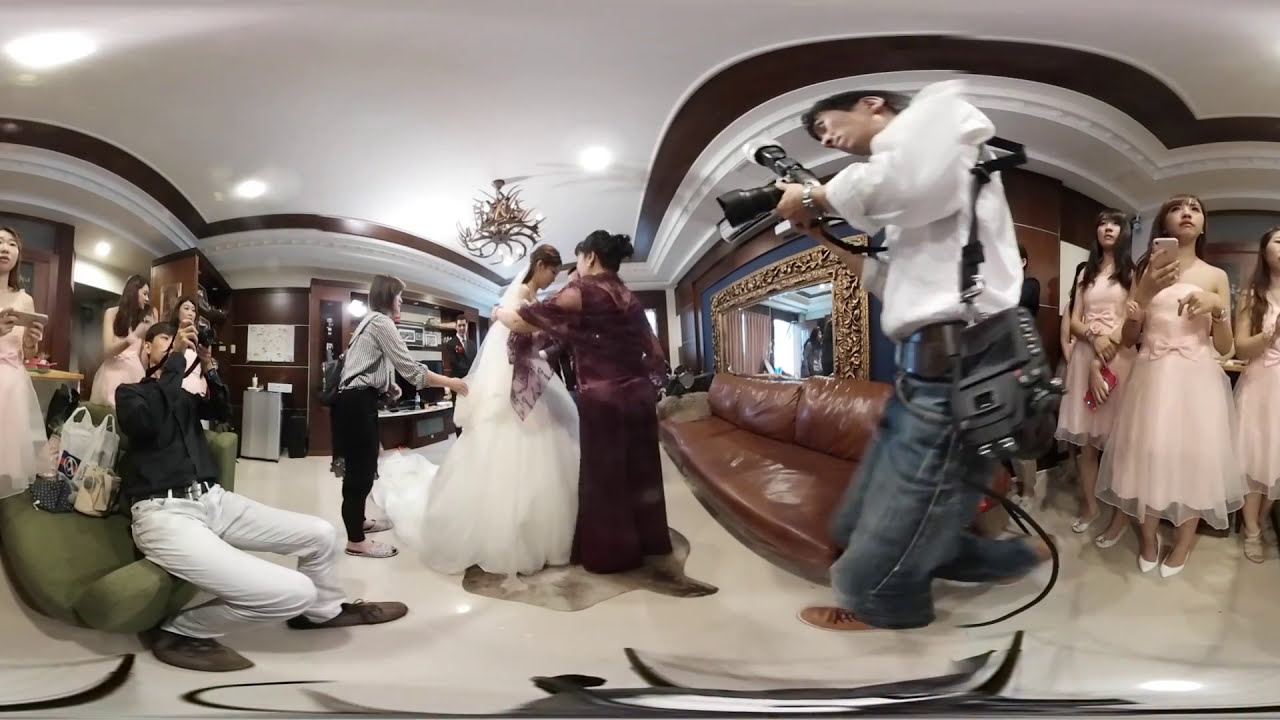This indoor fisheye lens photograph captures a lively moment from an Asian wedding preparation. Central to the image is the bride, adorned in a voluminous white wedding gown with a trailing veil and sporting dark brown hair, her head bowed slightly to the right. Attending to her is a lady in a maroon silk dress with a shawl, likely offering support or adjustments. Behind the bride, another woman with short brown hair in a white long-sleeve shirt and black slacks is carefully arranging the bride's veil.

To the right stands a professional photographer dressed in blue jeans and a white shirt, equipped with an extensive array of black camera gear, ready to capture the moment. Surrounding him are three bridesmaids in off-shoulder light pink dresses, holding phones and purses, blending into the bustling scene.

On the left side of the image, a man in a black shirt and white slacks is seated on a green couch, aiming his camera upwards, presumably to document the occasion. Adjacent to him, more bridesmaids in pink dresses add to the vibrant atmosphere.

The room's decor includes a brown leather couch positioned centrally, a gold-framed mirror above it, blue walls, and a white ceiling with brown trim. The distorted effect of the fisheye lens accentuates the room's rounded structure, creating an intriguing visual interplay that stretches and compresses the scene's elements, emphasizing the bride and her attendants while playfully warping the surrounding figures and furniture.